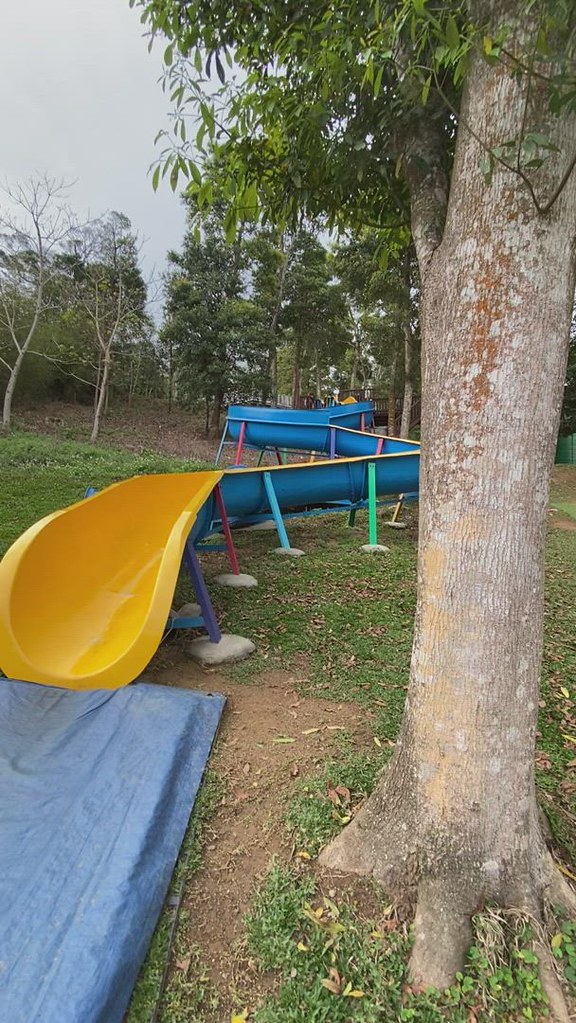This detailed colour photograph, captured in a portrait orientation, depicts a vibrant outdoor scene at what appears to be an adventure or water park. Dominating the left foreground is the exit of a twisting slide, which is distinctly industrial in design. The slide's exterior is a pastel blue and its interior a bright yellow, sinuously snaking backwards to the right, then curling left, and right again, eventually disappearing from view, seemingly descending out of sight. The slide is supported by an array of colorful metal struts—featuring hues of purple, reddish-pink, light blue, and green—secured by roughly shaped concrete bases. 

A prominent tree trunk rises out of the frame on the right, with green foliage visible at the top. The entire scene is bathed in natural light that highlights the lush green grass beneath the structure. Positioned at the slide's exit, a blue mat is observable, designed to cushion the landing of individuals emerging from the slide. This detailed setup suggests a well-manicured park space, complete with vegetation and large outdoor structures.